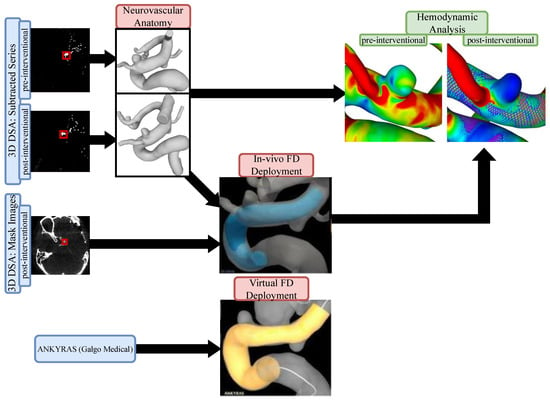The image presents a complex diagram of neurovascular anatomy and hemodynamic analysis, likely intended for medical students or professionals. On the left, the diagram features a vertically aligned section with three black-bordered boxes labeled "3D VSA Substructed Series" and "3D VSA Mask Images." These boxes contain intricate white and red structures, resembling medical imaging results, possibly X-rays, that appear to show neurovascular details. Arrows connect these boxes to two other sections labeled "NVOFD Deployment" and "Virtual FD Deployment," which display tubular structures in yellow and blue against dark backgrounds. Additionally, a section at the top, labeled "Hemodynamic Analysis," includes two images with infrared-like color schemes of reds, greens, and blues, likely illustrating blood flow or pressure variations. The diagram includes annotations for "pre-interventional" and "post-interventional" stages, indicating changes before and after a medical intervention. Overall, the detailed layout with multiple color-coded boxes, connecting arrows, and descriptive labels showcases various aspects of neurovascular imaging and procedural analysis.